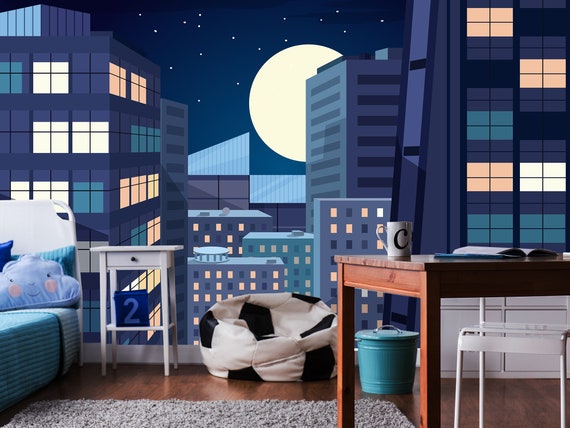The image depicts the cozy interior of a bedroom, likely designed for a young individual. Dominating the scene is a feature wall adorned with wallpaper that mimics a city skyline at night, characterized by tall buildings in dark navy hues with illuminated windows. A prominent round moon, partially obscured by a skyscraper, captivates the viewer's attention.

On the right side of the room stands a wooden desk, accompanied by a white chair. The desk is neatly arranged with an open book and a coffee mug bearing the letter 'C'. Nearby, a small teal trash can is positioned against the wall, beside a playful beanbag chair designed to resemble a soccer ball.

To the left, there is a glimpse of a white bedside table, and further left, part of a bed is visible. The bed features a white headboard and blue bedding, accented with a cloud-shaped pillow, which has a happy face. Additional details include a light blue bucket near the beanbag, and a soft rug that covers portions of the floor, with natural light filtering in from a window on the far left. The decor and layout suggest a youthful and inviting living space.